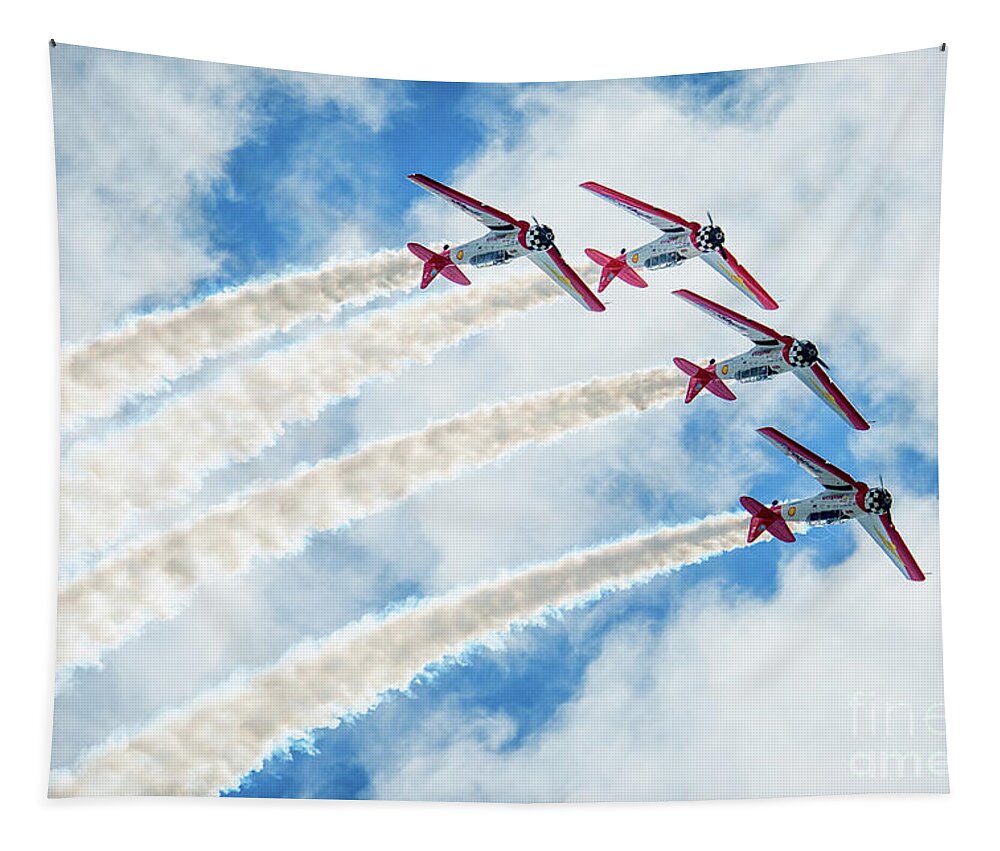The image is a detailed tapestry pinned up by thumbtacks in the upper left and right corners, depicting an aerial display. The backdrop of the tapestry is a vibrant blue sky adorned with fluffy white clouds. Central to the tapestry are four red and white propeller planes flying in a close and precise upside-down formation, reminiscent of an air show or wartime aerial maneuvers. Each plane is uniform in appearance, featuring distinctive black and white checkerboard patterns near their propellers. These planes are trailing streams of smoke behind them, enhancing the dynamic and lively depiction of their flight.